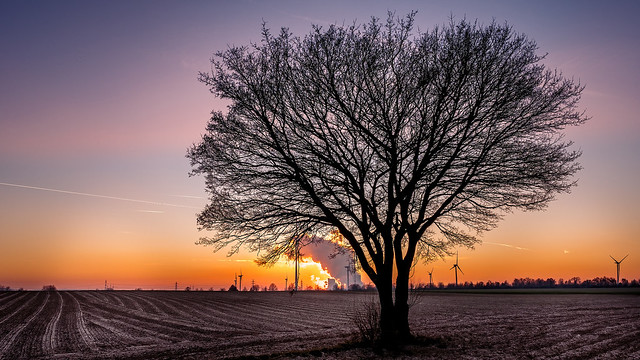In this beautifully composed rectangular photograph, we observe a tranquil yet evocative scene of a large, tilled farm field during either late fall or winter, characterized by the absence of snow on the ground. Dominating the center of the image stands a solitary, silhouetted tree, its branches devoid of leaves, suggesting a dormant period. The tree's trunk splits into two prominent sections early on, giving it a distinctive shape. The field surrounding the tree is crisscrossed with various tire tracks, adding texture to the earth.

The sky paints a dramatic backdrop with layers of color: a deepening blue or light purple occupies the upper half, transitioning into a vibrant reddish-orange near the horizon, indicating that the photo was taken at dusk, with the sun not quite below the horizon yet. Backlit, the tree appears almost black and shadowy against the glowing sky.

Prominent in the horizon, a large plume of white smoke rises, likely from an industrial source such as a factory or power plant, reinforcing a juxtaposition between nature and industry. Similarly, multiple large wind turbines, backlit by the remaining daylight, dot the horizon to the right of the tree, their blades barely visible but defining their presence as instruments of power generation.

The overall scene exudes a cold, serene ambiance, perhaps reflective of a typical prairie landscape in the United States, possibly a place like Nebraska. The combined elements of the setting sun, the shadowy tree, industrial smoke, and wind turbines create a striking, contemplative image of rural life intersecting with modern industry.